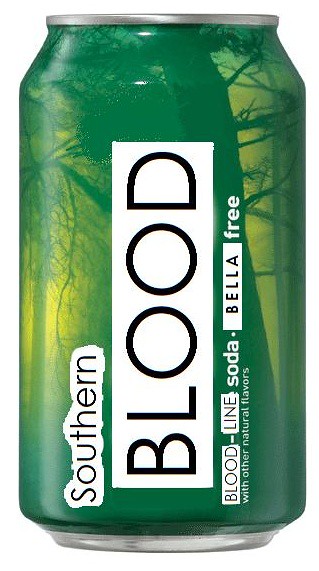The image features a close-up of a soda can meticulously cut out against a completely white background, resembling a professional Photoshop edit. The can itself is predominantly green, emblazoned with various shades of green and a design that includes tree trunks and branches, which stretch diagonally from the bottom right to the top left at an 11 o'clock angle. This background gives an eerie swamp-like appearance with gaps between the lime-yellow tree trunks and smaller branches. The can's top and bottom edges are silver, adding a traditional can-like finish.

The text on the can is oriented vertically, requiring a 90-degree anticlockwise turn of the head to read. The brand name "Southern Blood" is prominently displayed, with 'Southern' in smaller letters and 'Blood' in large, black letters encased in white rectangles. Below this, "bloodline soda" is broken up into segments: "blood-" in black text on a white rectangle, "line" in black text without a rectangle, and "soda" in white text. Further down, it reads "Bella-free," broken into "Bella" in bold black text within a white rectangle and "free" in black text outside any rectangle. Additionally, it mentions "with other natural flavours," implying that the soda is marketed as a healthier, more natural option, despite not specifying the actual flavor.